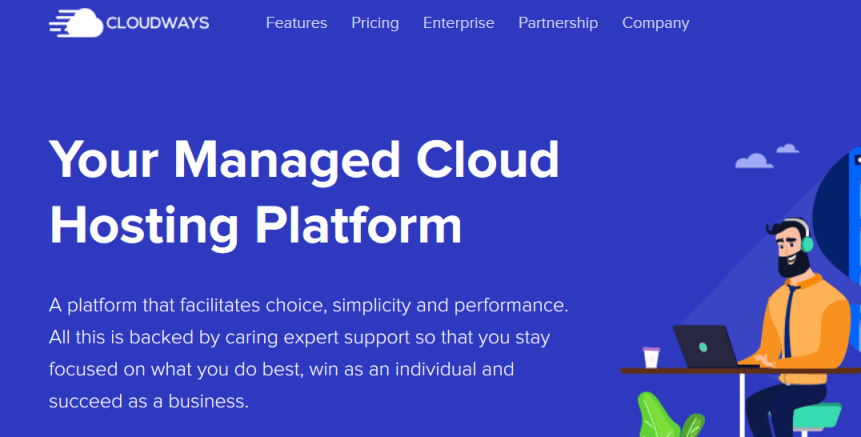The image is a screenshot from a desktop view of a website with a dark blue or purple background. At the top left, the Cloudways logo is prominently displayed. The top menu bar contains several options, including "Features," "Pricing," "Enterprise," "Partnership," and "Company." The central headline text reads: "Your Managed Cloud Hosting Platform." Below this, a subheading describes the platform as facilitating choice, simplicity, and performance—all bolstered by expert support so users can stay focused on their core tasks, whether aiming to win as an individual or succeed as a business.

To the right of the text, there is a graphic illustration of a man working at a table with a laptop. He is wearing an orange shirt paired with a dark purple tie and has a beard. The man is also wearing headphones while seated on a green stool. Underneath the table, there is a plant, and on the table, there's a drink.